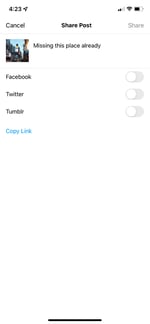A blurry screenshot of an Instagram post-in-progress is displayed. The top left corner indicates a time of 4:23, with location services enabled. The status bar shows icons for battery life, wireless connection, and cellular signal strength. Central to the image are options for "Next" and "Cancel," with a bold "Share Post" label flanked by a lighter "Share" option on the right.

A thin gray line separates the menu from a preview of the image to be shared, accompanied by the caption "Missing this place already." The image itself is indistinct, but it appears to feature Times Square. Beneath the photo, toggles for sharing on Facebook, Twitter, and Tumblr are all turned off. A blue "Copy Link" hyperlink is visible below these options. At the bottom of the image, the swipe bar for closing the app is faintly visible.